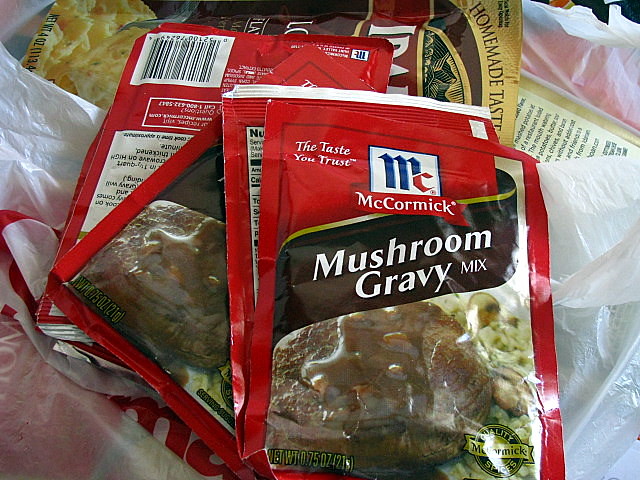In this detailed photograph, a grocery bag containing several packets of instant food products is displayed on a surface. The grocery bag, which is loosely folded around its contents, prominently features a red logo with the word "elm". At the top of the assortment, centrally positioned, is a packet of McCormick Mushroom Gravy Mix, emblazoned with the phrase "The Taste You Trust" in bold red lettering. Underneath the McCormick packet, a portion of a brown packet from the Idaho brand, known for its homemade taste, is visible. Additionally, the back of another unidentified packet peeks out from beneath, hinting at more items tucked away within the bag.